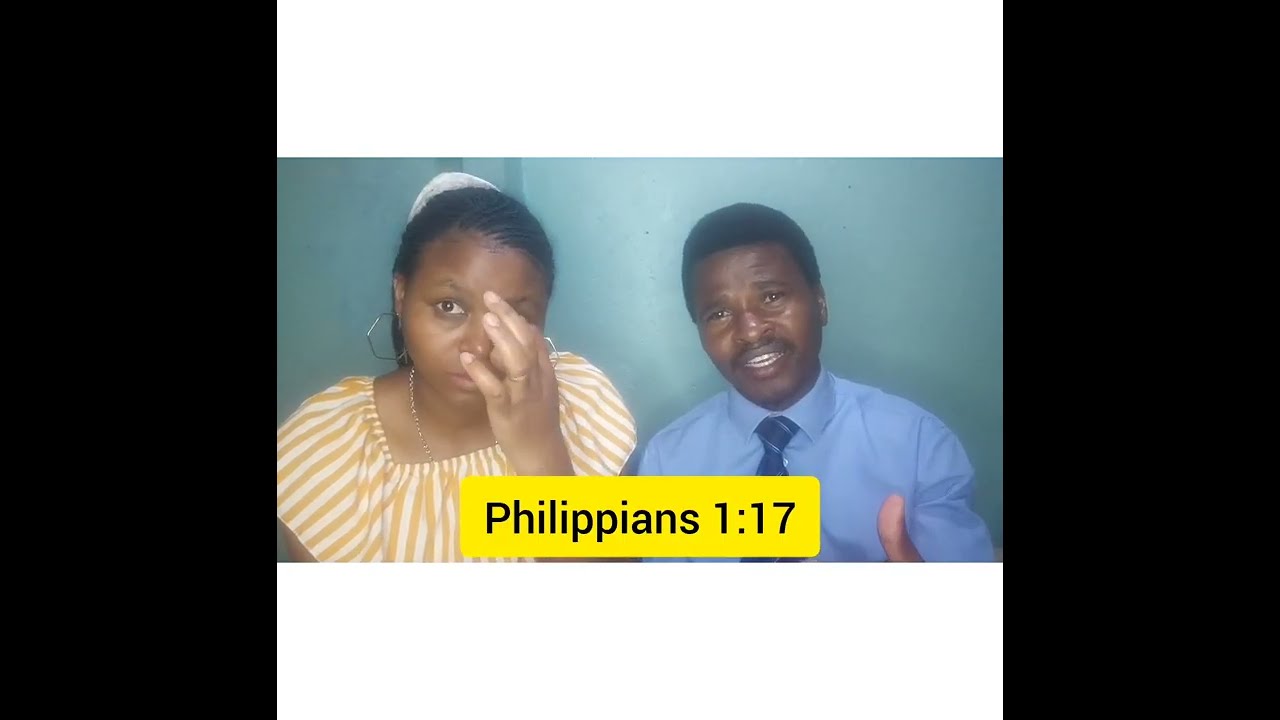In this detailed image, two black individuals are engaged in a video call. On the right side, a man is dressed in a light blue dress shirt paired with a navy blue tie. He has short black hair and a mustache, with his head slightly tilted to the left, displaying an expression of shock or disbelief. On the left side, a woman wears a white and orange-striped dress, accessorized with a thin gold necklace, large round earrings, and a black hairband that holds her hair back. She appears to be wiping a tear from her face. Below them, in a yellow rectangle with black text, is the scripture reference "Philippians 1:17." The image is bordered by large white bars at the top and bottom and black bars on the sides, creating a framed effect. The background behind them is a plain light green wall, likely part of the video call setting.